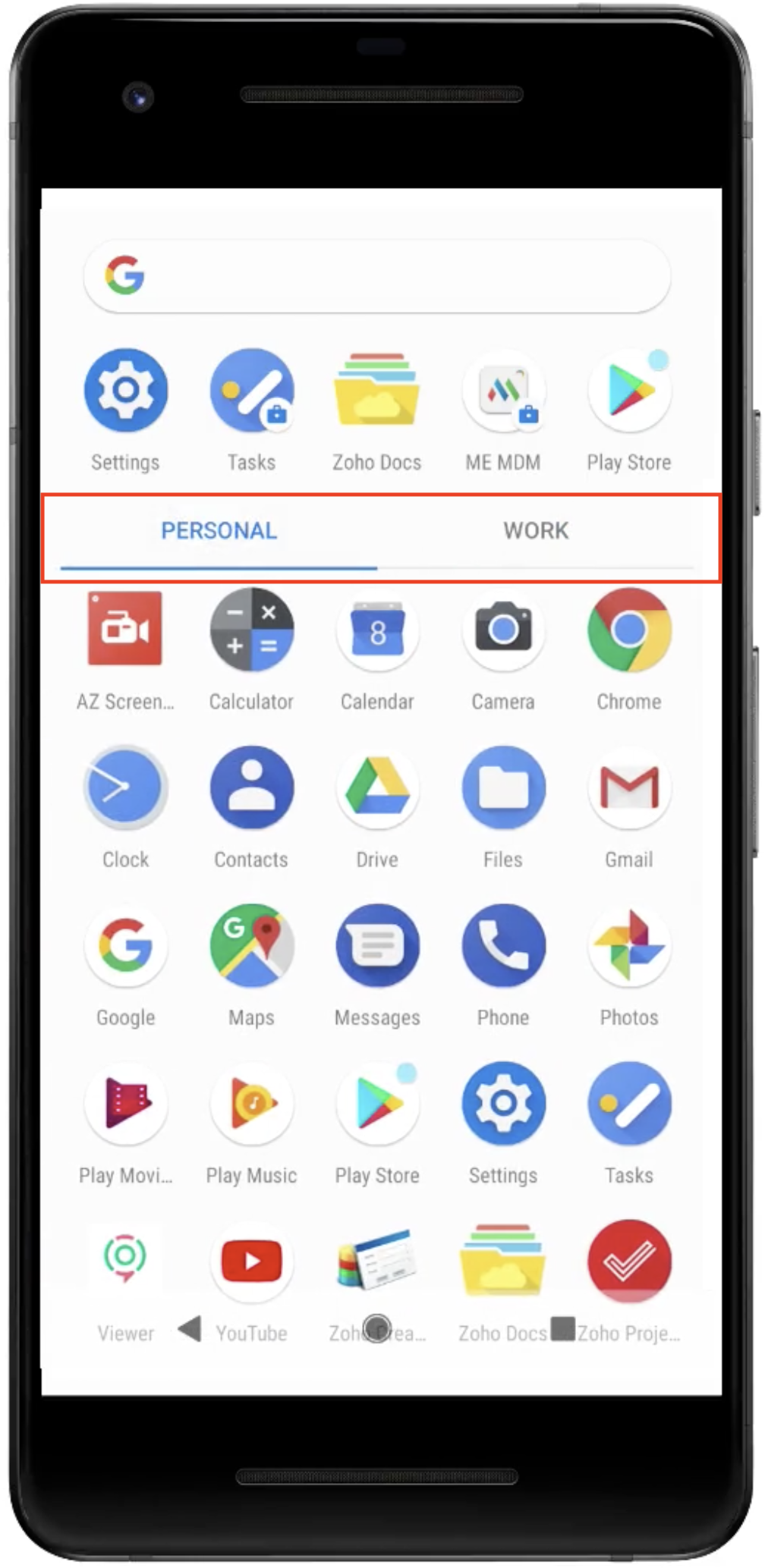The image portrays an older Android smartphone encased in a gray protective cover. The device features distinct black bezels at both the top and bottom, with buttons on the side including a smaller button, likely the power button, above a larger volume control.

The screen displays a white background with the Google search bar at the top. Below this, various app icons are visible, organized in rows. These include:

- Settings
- Tasks
- Zoho Docs
- MEMDM
- Play Store
- A highlighted section titled "Personalized Work," where "Personalized" is blue and underlined, and "Work" is in gray and outlined in red.

Additional app icons listed are:

- Add Screenshots
- Calculator
- Calendar
- Camera
- Chrome
- Clock
- Contacts
- Drive
- Files
- Gmail
- Google
- Maps
- Messages
- Phone
- Photos
- Play Movies
- Play Music
- Play Store
- Settings
- Tasks
- Viewer
- YouTube
- An unreadable app starting with 'Z'
- Zoho Docs
- Zoho Projects

At the very bottom of the screen are the Android navigation buttons: a back arrow (triangle), home button (circle), and a recent apps button (square). 

The phone interface provides a clear and organized view of the user's frequently used applications, emphasizing its functionality and user customization options.